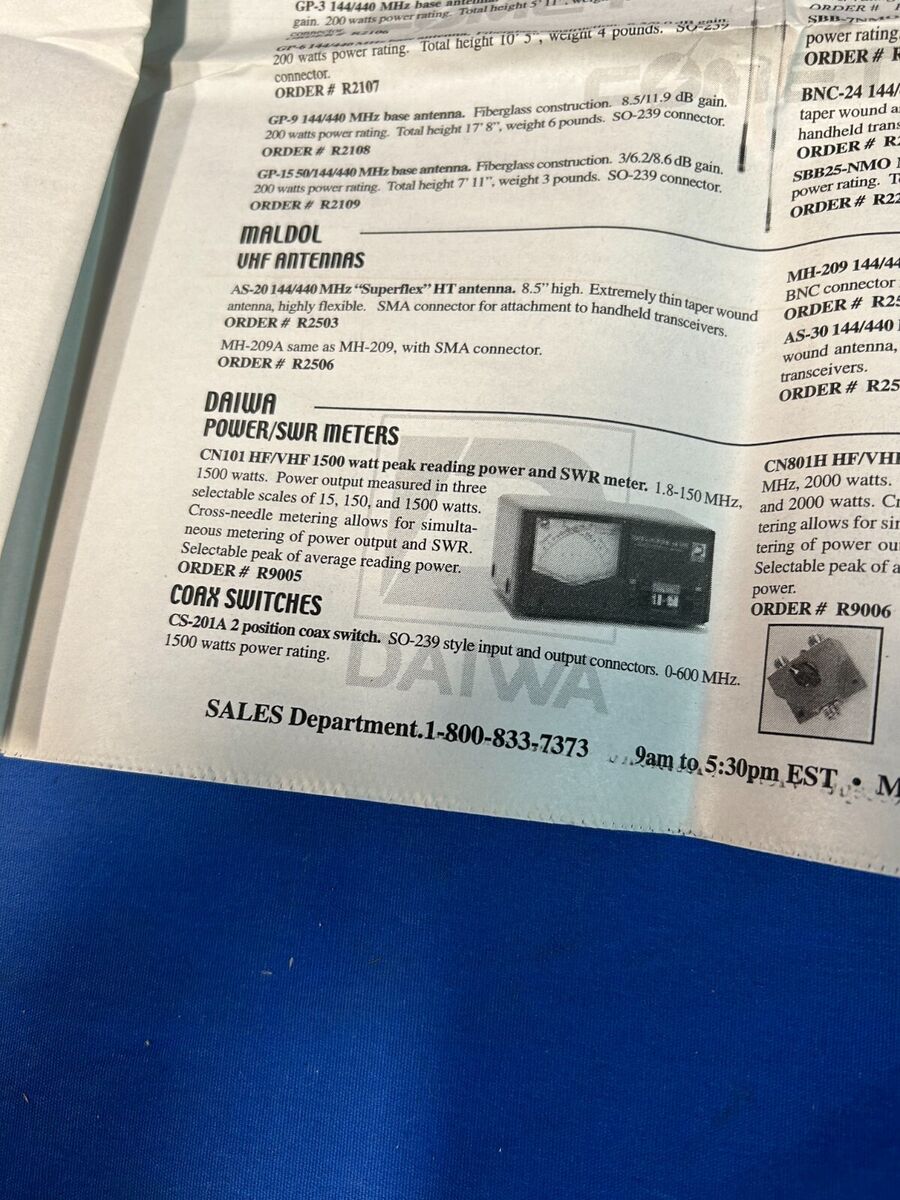This color photograph depicts a section of a black-and-white newspaper, possibly a flyer for an electronics store, against a blue background. The slightly tilted and creased white paper holds detailed listings and descriptions of various electronic devices and components. The central listing features a small photograph of a Daiwa Power/SWR meter, model CN-101, capable of 1500-watt peak reading power. It measures power output in three selectable scales of 15, 150, and 1500 watts and uses cross-needle metering for simultaneous metering of power output and SWR. The order number for this device is R9005. Below it is a listing for coax switches, specifically the CS-201A two-position coax switch with SO-239 style input and output connectors, supporting 0 to 600 megahertz and a 1500-watt power rating. Also featured is a listing for Maldol VHF antennas, specifically the SuperFlex HT antenna, which is 8.5 inches high, highly flexible, thin taper wound, and includes an SMA connector for hand-held transceivers, with the order number R2503. The sales department contact information is listed at the bottom, with the phone number 1-800-833-7373, operational from 9 a.m. to 5.30 p.m. Eastern Standard Time. The right side column of the paper is partially visible, but its text is largely cut off.